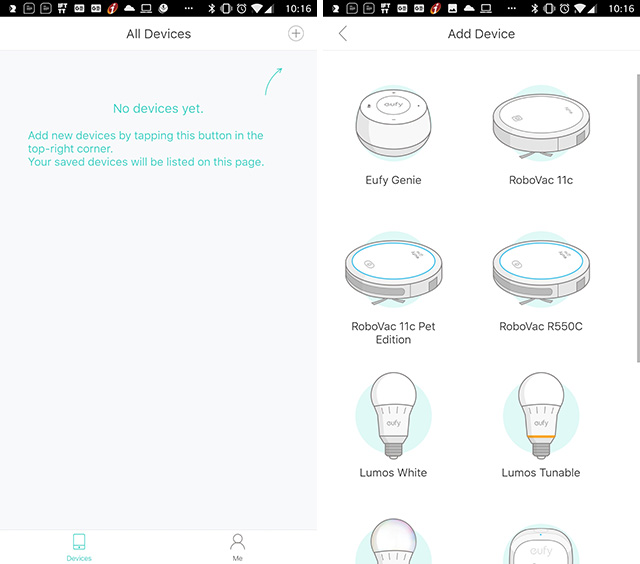**Detailed Caption:**

This image consists of two screenshots from a mobile app, presented side by side against a white background. 

**Left Screenshot:**
The left screenshot displays a section titled "All Devices" at the top. In the top-right corner, there is a plus button (+). Below the title, the screen body contains text in blue that reads, "No devices yet. Add new devices by tapping this button in the top right corner." An arrow points towards the plus button to emphasize where users need to tap to add new devices. The overall interface is minimalistic, making it clear that no devices have been added yet.

**Right Screenshot:**
The right screenshot shows the "Add Devices" section, where users can add new devices to the app. This screen displays sketches of household items, primarily small electronics, organized in a grid format.

- **First Row:**
  - An icon labeled "Eufy Genie."
  - An icon labeled "RoboVac," showing a circular vacuum cleaner.

- **Second Row:**
  - Two variations of the "RoboVac," again depicting circular vacuum cleaners.

- **Third Row:**
  - An icon labeled "Lumos White," representing light bulbs from Eufy.

The bottom row of the screen has been cut off, and the total number of items in this screen could be six, nine, or eight. Both screenshots feature a white background.

**Top Bar Elements:**
At the very top of both screenshots, there's a black stripe displaying phone-related icons such as signal strength, Wi-Fi, battery status, and the time, which is shown as 10:16 on the top-right corner. 

This dual-screenshot setup provides a comprehensive view of the current 'no devices added' state and the options available for adding new smart home devices within the app.